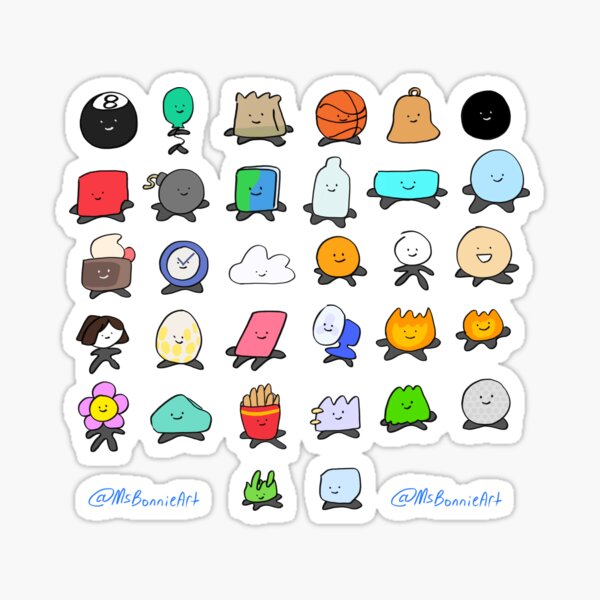This image showcases a delightful collection of 32 graphic art stickers set against a light gray background. Arranged in a 6x5 grid with two extra stickers at the bottom, these adorable cartoons are neatly placed on a white background which contrasts beautifully with the pale blue backdrop. Each sticker features a playful, cartoony style, all adorned with expressive little smiley faces. 

Among the diverse array of characters, you’ll find an eight-ball, a basketball with feet, a merry little bell, a whimsical campfire, and even a cheerfully steamy cup of coffee. Other endearing figures include a golf ball, a container of french fries, an egg, a lightbulb, a milk carton, a bomb, a clock (which looks slightly frowny due to its clock hands resembling eyebrows), and even a character that looks like a slime from the Dragon Warrior series. There’s also a representation of common objects like a box of fries, a flower, a red square, a cloud, a book, and a toaster.

Accentuating the whimsical charm of these stickers, the artist, identified as @MsBonnieArt, has their tag handle displayed in blue text at both the lower left and lower right corners of the image. The vibrant characters benefit from a simple coloring technique without much shading, and their bright, varied hues further enhance the cute aesthetic. This charming set of stickers is sure to be a hit with children and anyone who appreciates playful, imaginative art.